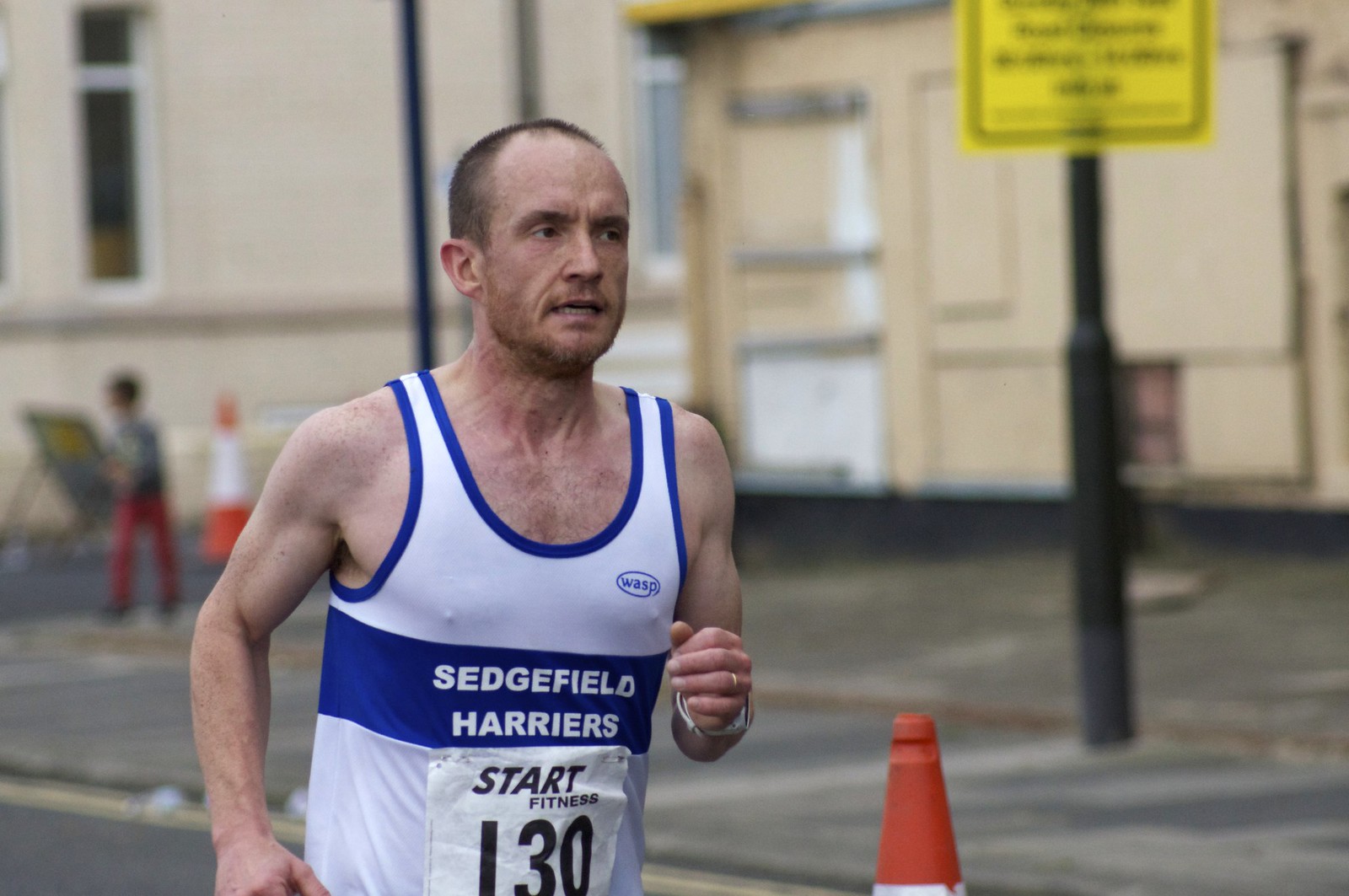This detailed image captures a focused, light-complected male runner, likely in his late 40s, participating in a marathon. He is sporting a blue and white tank top displaying a circular emblem with the word "Wasp" and the name "Sedgefield Harriers" across his chest. Below these identifiers, his race bib reads "Start Fitness 130." He wears a ring on his left-hand ring finger and a smartwatch, indicative of his commitment to tracking his performance. His shaved head and receding hairline are noticeable, along with his tired yet determined expression. The background is blurred, highlighting the runner's concentration, but you can glimpse older yellowing buildings, a large yellow signpost, and orange and white parking cones. To the back left, a person appears to be painting, adding a layer of everyday activity to the race scene.